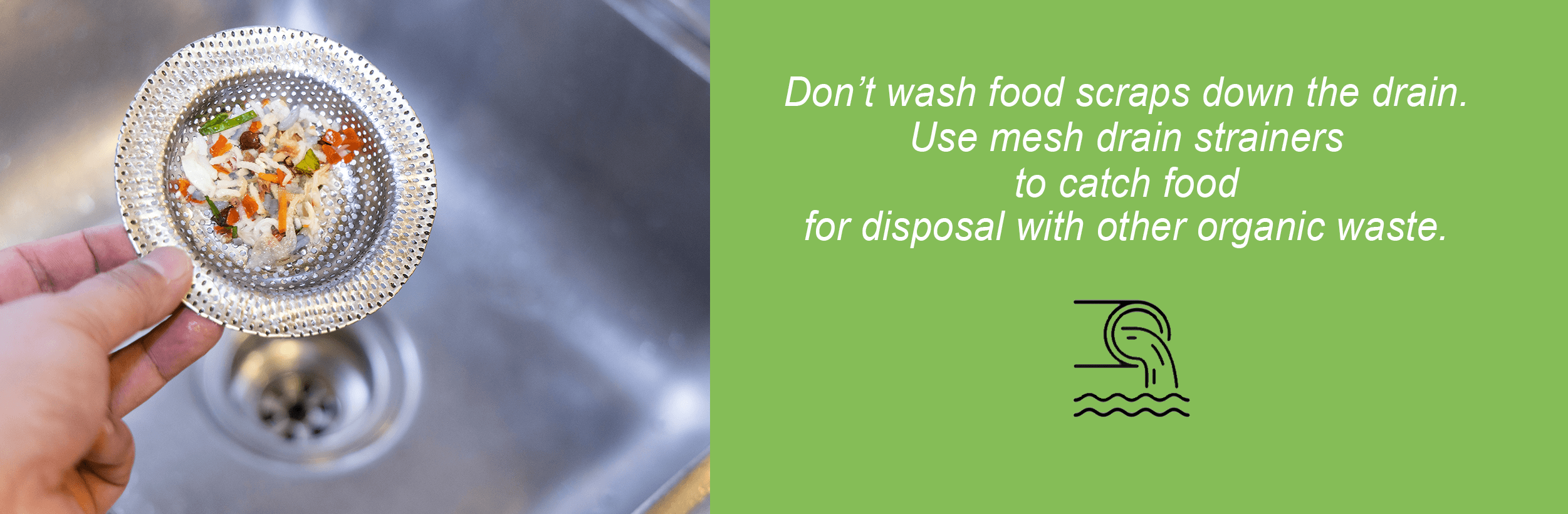The image is a promotional ad likely from a municipal water department, emphasizing the importance of using mesh strainers to catch food scraps and prevent them from going down the drain. On the left side of the image, there is a color photograph of a stainless steel sink with a drain covered by a silver mesh strainer. A Caucasian hand, using the thumb, index, and middle fingers, holds the strainer, which is filled with various food scraps including bits of orange, green, red, and potentially pieces of peppers, pasta, and rice. The background of the sink is also visible, showcasing its metallic interior. 

On the right side, against a lime green background, white text reads: "Don't wash food scraps down the drain. Use mesh drain strainers to catch food for disposal with other organic waste." Below this message, a small black drawing depicts a pipe discharging water into what appears to be a lake or stream. This detailed graphic reinforces the environmental message by illustrating the consequences of food scraps entering the wastewater system.